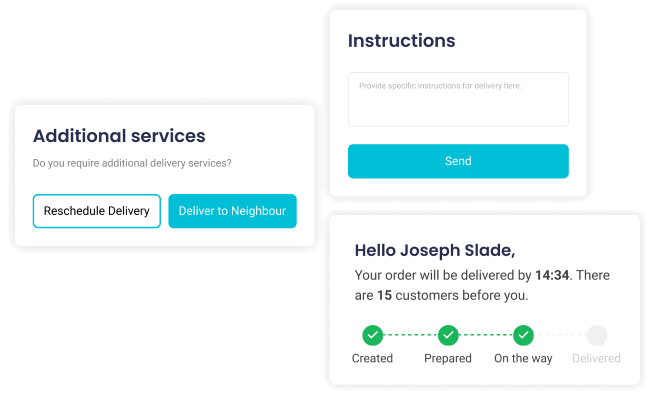The image is a snapshot resembling a disorganized webpage layout, with various elements scattered in a non-linear fashion. Key components include:

1. **Additional Services Section**: A bold header stating "Additional Services," followed by "Do you require additional services?" Below this, there are interactive buttons including "Reschedule Delivery" and "Deliver to Neighbor," both in a distinct blue color.

2. **Instructions Section**: Another segment titled "Please provide specific instructions for delivery here," accompanied by a blue "Send" button where users can presumably submit their instructions.

3. **Delivery Status Window**: A personalized message addressing "Joseph Slade," indicating that his order is scheduled for delivery at 14:34. It further notes that there are 15 customers ahead of him in the delivery queue.

The overall image suggests that Joseph Slade has made an order with a service allowing delivery rescheduling, specific delivery instructions, and real-time updates on his order status. The scattered placement of these elements gives the appearance of a disrupted or unfinished webpage.